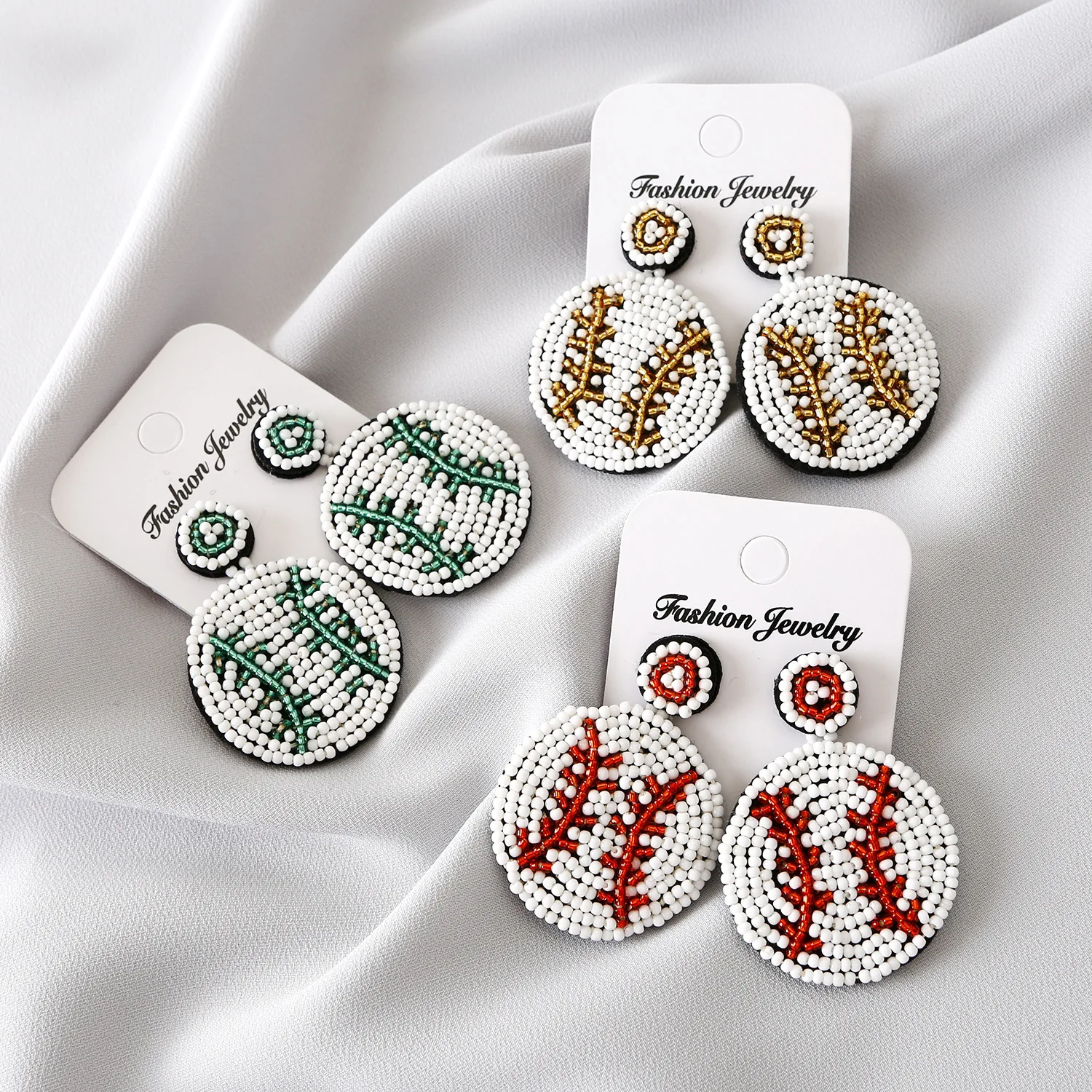In this image, three sets of earrings, resembling baseballs due to their stitching pattern, are displayed. Each set features a circular design with variations in the stitching color: the bottom right pair has classic red stitches, the center-left pair showcases teal stitches, and the top-right pair is detailed with gold stitches. All earrings are mounted on white cards marked with the words "Fashion Jewelry" in elegant black cursive. The cards rest on a textured, crumpled, white satin-like fabric, enhancing the soft and sheer appearance of the background. The earrings on the right stand upright, while the left pair is slightly tilted to the top left. These earrings, made of tiny beads on dark bases, offer a handmade aesthetic and are designed for pierced ears.